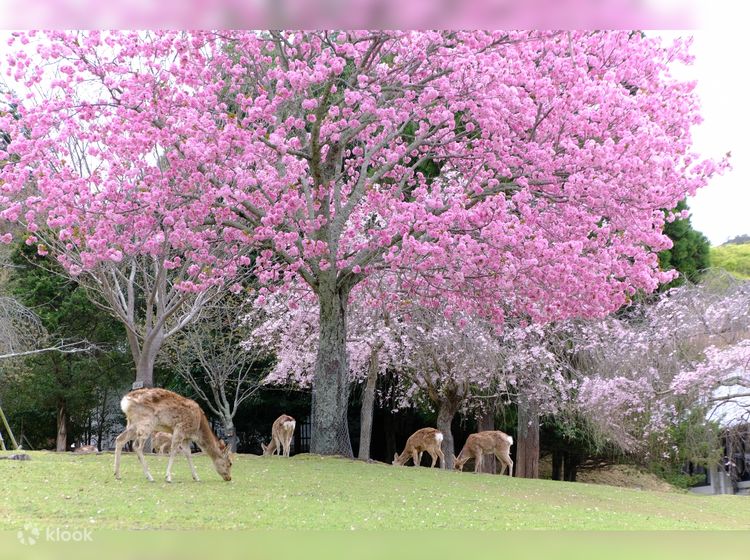The image depicts a serene garden scene, likely in Japan, characterized by a prominent tree with a brown trunk and vibrant pink cherry blossoms. Surrounding this central tree are additional trees with both bright and light pink blossoms, as well as some with lush green canopies. In the foreground, four brown deer with white tails are seen grazing on a soft shade of kelly green grass, all with their heads and necks bent down to eat. A black wrought-iron gate and a building can be observed in the background, subtly framed by the diverse array of trees. The bottom left-hand corner of the image features a logo that reads "KLOOK".